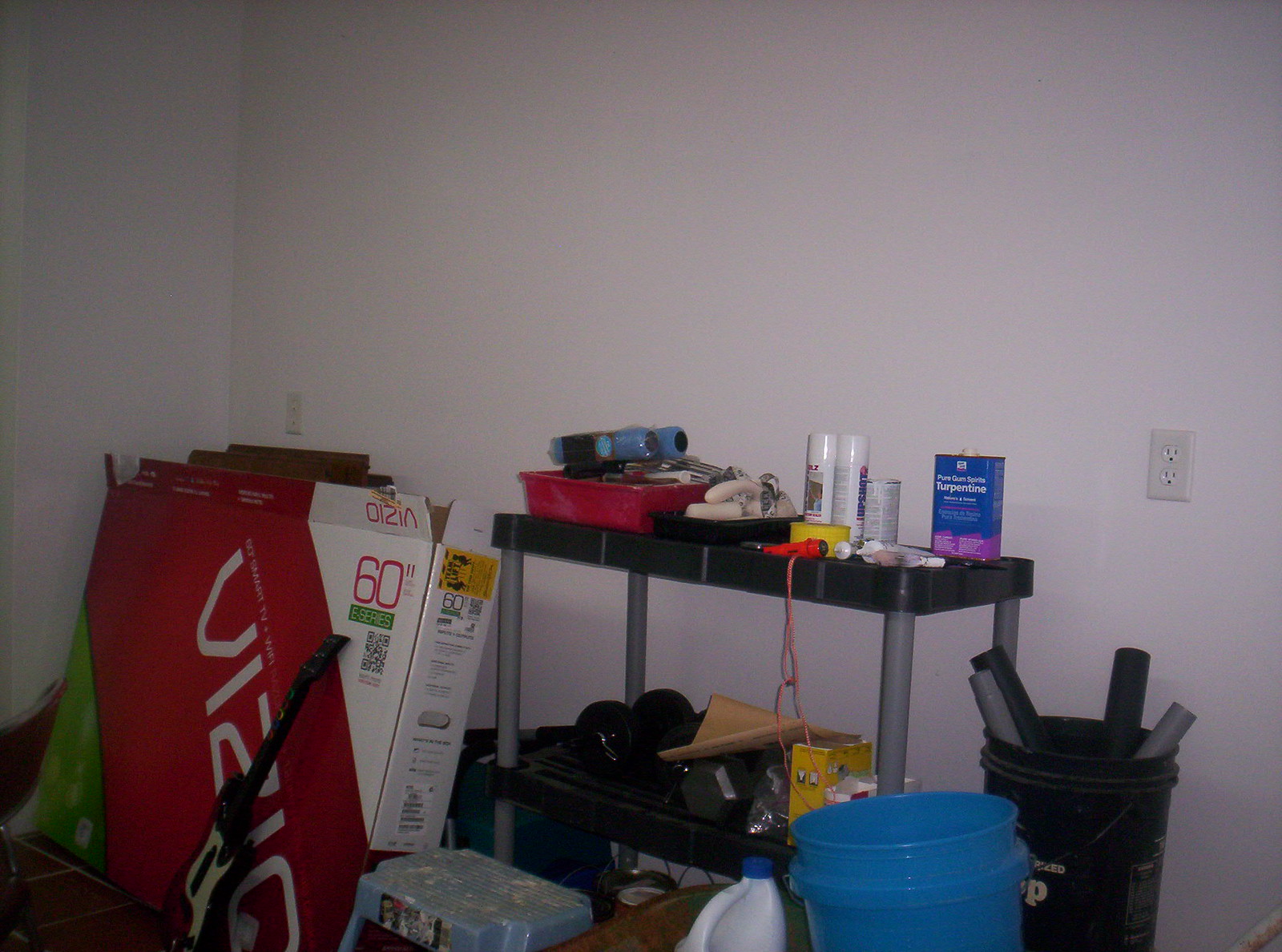The photograph depicts a cluttered and untidy room, characterized by a disorganized assortment of items piled atop one another. Dominating the scene is a large box for a Vizio television measuring 60 inches. Positioned beneath this is a small workbench cluttered with various tools and materials, including bottles of turpentine, cans of spray paint, rolls of tape, and various other tools and packaging. The workbench also features a lower shelf, which holds more of the same types of objects.

In addition, there are two black, indeterminate objects adjacent to the workbench, as well as a pair of weightlifting weights with a tan piece of paper resting on top. Flanking the workbench are two buckets: one blue and one black. The blue bucket appears empty, while the black bucket contains several gray and black styrofoam tubes. 

Beside the blue bucket, there is a container resembling a bleach bottle, although the label is not clearly visible. Near this, a heavily used blue step stool shows signs of extensive wear, with numerous markings covering its surface. All of these items are situated in the corner of a plain white room where two walls meet, with a power outlet visible on each wall. The walls appear undamaged and are bare, with no decorations or hanging items.